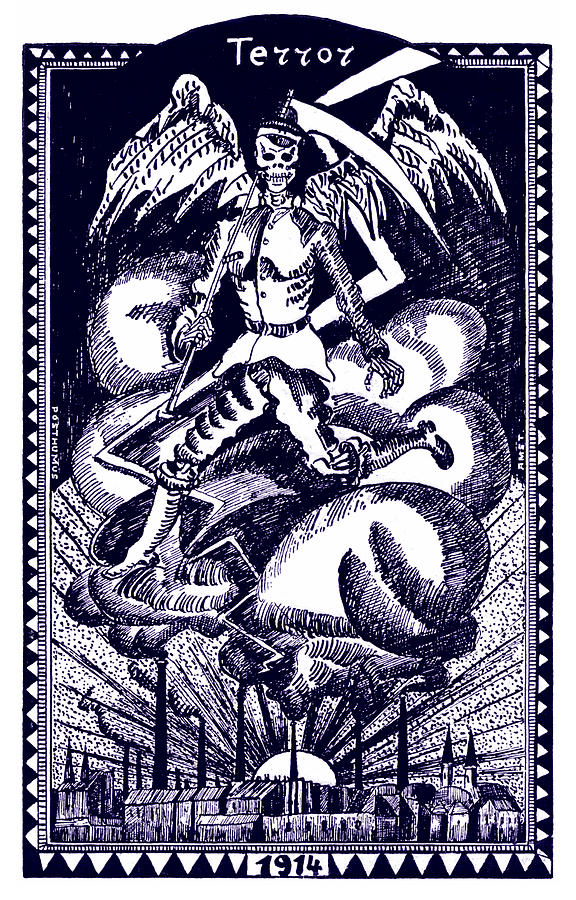The image is a monochromatic, rectangular poster with a black background and intricate borders featuring small white triangles along the edges. At the top, the word "TERROR" is prominently displayed in bold white letters, with a stylized and possibly reversed 'R'. Below this, a striking hand-drawn illustration dominates the center of the poster, portraying an ominous figure with a skeleton head. The figure is clad in a detailed outfit, including pants and a coat with large, ornate buttons and black stripes reminiscent of ribs. White, pointed feathers trimmed in black streaks form wings that rise dramatically from its shoulders.

The skeletal figure, wielding a sickle or scythe in its right hand, appears to be running or floating above a cityscape. The city's skyline is dotted with numerous pointed towers, steeples, and thin, straight trees. At the horizon, a semicircular sun is either setting or rising, casting speckled white rays with black stripes across the sky. Behind the figure, the background is filled with white clouds or billowing smoke marked with black indentations, adding to the scene's eerie atmosphere. The bottom border of the poster is inscribed with the year "1914," anchoring the piece in a historical context. The detailed elements and intricate design render this piece a compelling and visually arresting artwork.